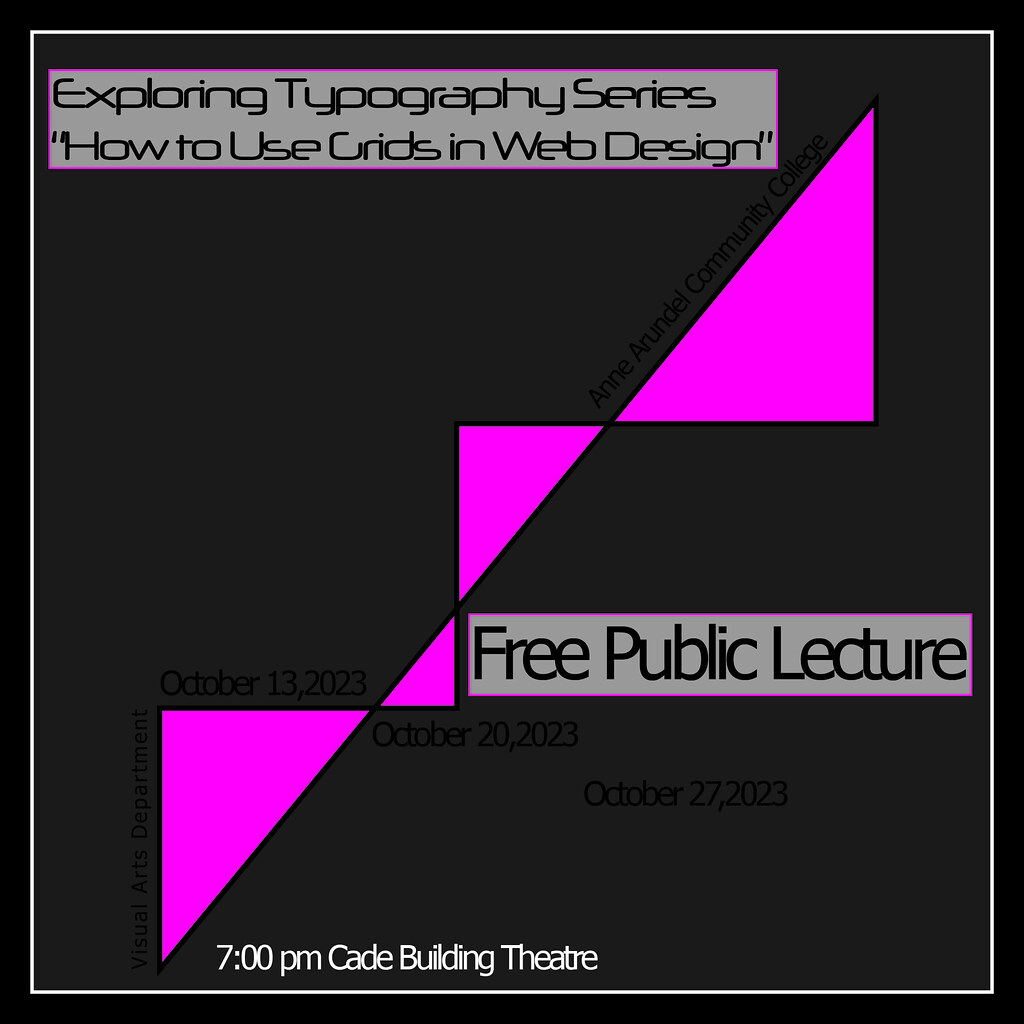The image is a graphic sign with a gray background bordered by a thin white square. In the center of this white border, there's a lighter gray square containing important information organized into two boxes. The text describes an event titled, "Exploring Typography Series: How to Use Grids in Web Design," clearly outlined in a red-bordered box situated at the top left. Beneath it, another red-bordered gray box announces, "Free Public Lecture." The graphic features four pink triangles: two larger ones positioned in the top left and right corners, and two smaller ones in the middle. Additional event details include the date, October 13th, 2023, and the location, Visual Arts Department, Anna Arundel Community College. A specific session is scheduled for October 27th, 2023, at 7 p.m., in the Cade Building Theater.